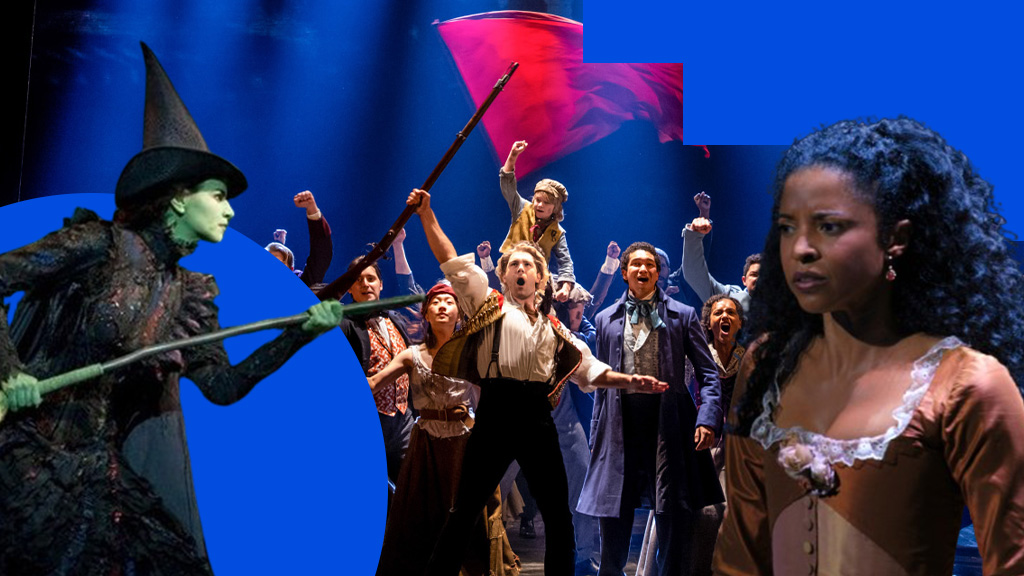In this vibrant image from a theatrical play inspired by "The Wizard of Oz," the scene features a dramatic encounter between key characters. On the left side of the stage, the iconic Wicked Witch of the West stands menacingly, adorned in her signature black outfit and triangular witch's hat, with her face painted a vivid green. Meanwhile, on the lower right, an African-American woman, potentially a modern take on Dorothy, looks contemplative and slightly bewildered, dressed in a light brown corset-like outfit. The center stage is dominated by an energetic, multi-colored ensemble of performers, some dressed in pirate-like attire, who seem to be either rising up or animatedly protesting. The backdrop is awash with hues of blue and red, contributing to the overall dynamic and theatrical ambiance. The rich color palette includes greens, blacks, blues, reds, browns, tans, whites, and beiges, harmoniously blending to create a visually striking scene.